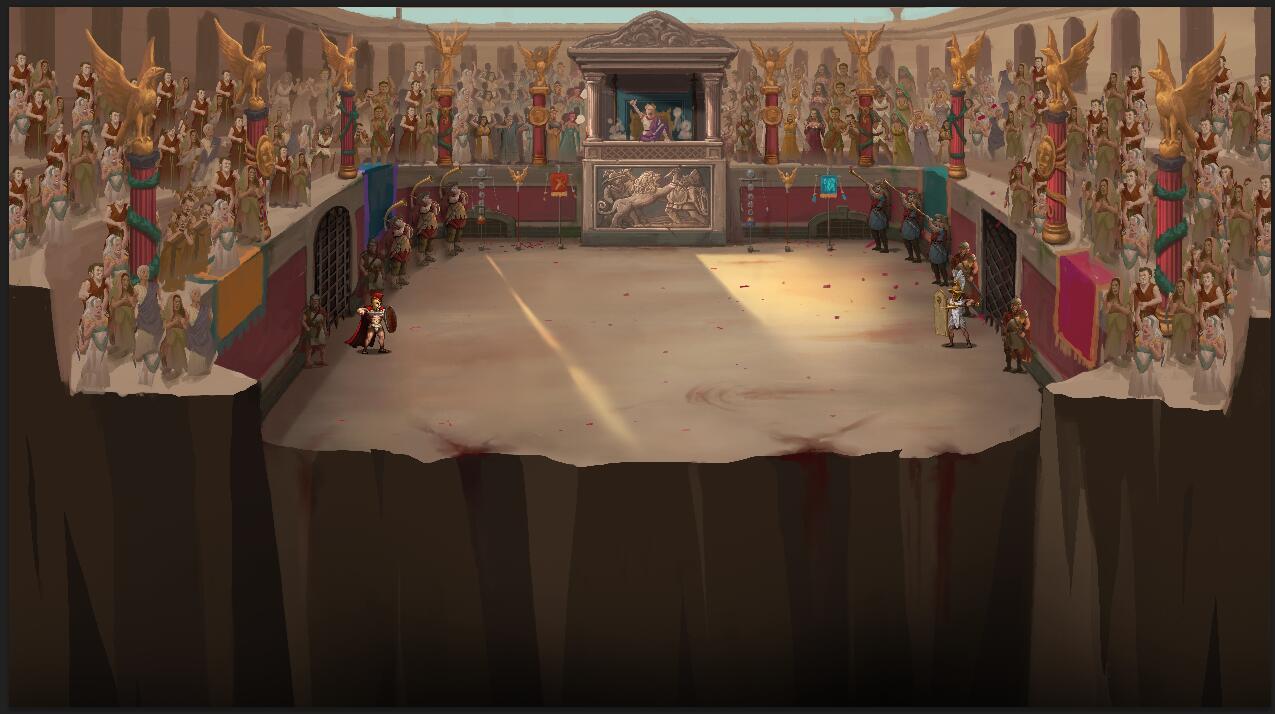The image appears to be a screenshot from a computer game, depicting a horizontally-aligned rectangular scene. At the bottom, vertical streaks of dark brown suggest the side of a cliff or a massive wall, forming the backdrop for a flat, tan-colored platform resembling a fighting arena. The arena is flanked by two opposing groups: on the left, three figures in red and gold, and on the right, three figures in blue, black, and green. These figures, although distant and lacking in clear detail, are blowing into musical instruments.

In the foreground, two primary fighters are positioned on opposing sides. The fighter on the left is distinguished by a red cloak, red hair, and a shield, while the fighter on the right is dressed in white with a gold hat and also equipped with a shield. The background features grandstands filled with spectators, all focused intently on the imminent combat.

On the upper tier of the structure, pink pillars wrapped in green and blue support golden bird statues atop red bases, contributing to the grandiose, castle-like ambiance of the arena. Two gated openings on either side hint at the possible release of additional participants or creatures into the arena. This colorful and dynamic scene, with its vivid reds and browns, suggests a gladiatorial event reminiscent of Roman times, primed for an epic showdown.